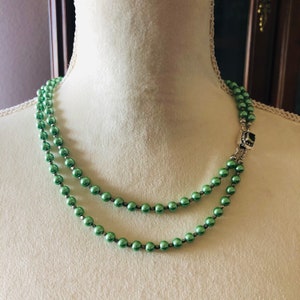The image features a close-up of a mannequin's neck and upper chest, which is covered in a felt or nylon-type material with visible seams running down each side. The mannequin is adorned with a green beaded necklace that consists of two strands, resembling Mardi Gras beads but shorter. These beads are shiny and of a jade or valuable stone appearance. The necklace is held together by a clasp located on the side of the neck, which is gold with a black stone in the middle and silver hoops connecting to it. The background of the image shows a brown wall with light tan or yellowish panels, and possibly a handle or fixture visible at the top. There are no other items, text, numbers, or words present in the scene. The display might be set in a women's clothing store or a museum, featuring colors such as green, brown, silver, gold, and off-white.